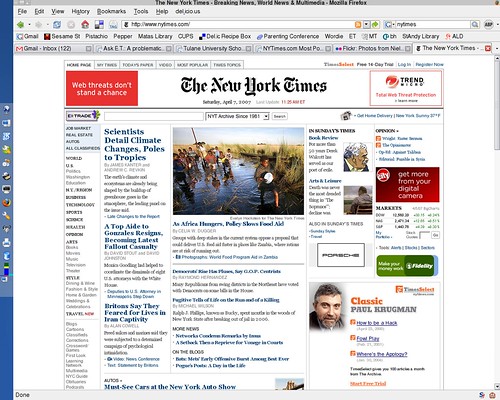This image is a screenshot of a New York Times webpage, resembling a window screen. The view includes a sidebar with a vertical blue bar featuring various program icons. Centrally, there's a large gray window that displays the New York Times content. At the top, the header reads "The New York Times" followed by sections like "Breaking News," "World News," and "Multimedia." It indicates usage of the Mozilla Firefox browser with numerous tabs open. 

The central feature is the newspaper's main page, with "The New York Times" prominently displayed in the center beneath which is the date, "Saturday, April 7, 2007," indicating the image's age. In the upper left corner, a red box advertises, "Web Threats Don't Stand a Chance," while another advertisement occupies the upper right corner.

Below the main title, a series of headlines are listed, including:
- "Scientists Detail Climate Changes, Polls to Tropics"
- "Top Aid to Gonzales Resigns, Becoming Latest Fallout Casualty"
- "Britain Say They Feared for Lives in Iran, Captivity"

This detailed screenshot either depicts an older browser session or someone accessing an archival edition of The New York Times online.